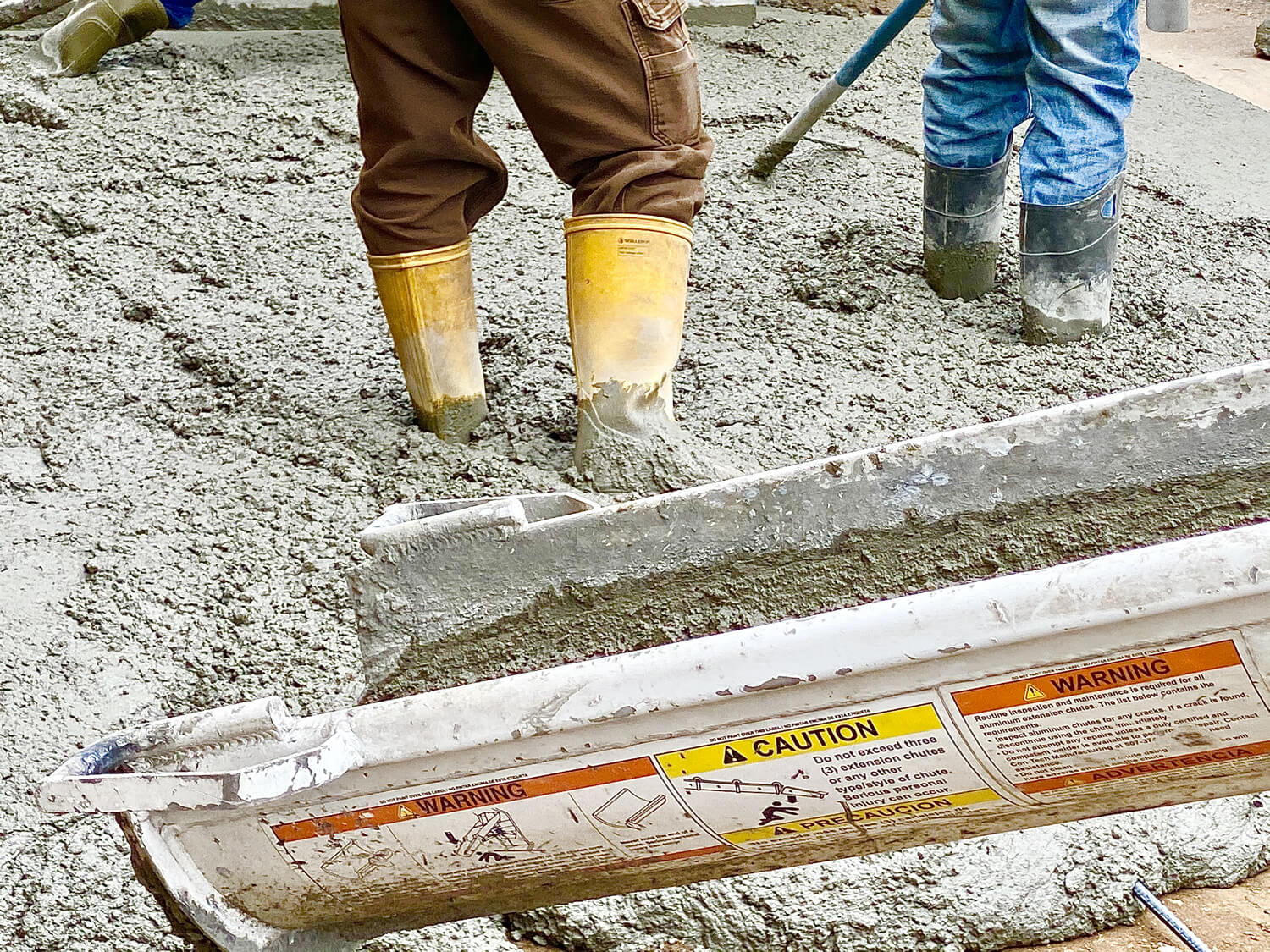In the image, two individuals are standing on freshly poured wet concrete, ready to smooth it out. In the foreground, there is a grey chute adorned with three distinct warning labels. The first label is orange with black text that reads "WARNING," accompanied by a black and white drawing. The second label features a yellow triangle with an exclamation mark inside, the word "CAUTION" in black, and a black and white depiction of a person kneeling. The third label has an orange banner at the top, a yellow triangle with an exclamation mark, and black lettering that reads "WARNING," followed by additional black text below. The individual on the left is wearing orange boots and brown pants, while the person on the right is dressed in blue jeans and grey boots, and is holding a blue and white pole. The scene captures a moment of teamwork and caution in a construction setting.